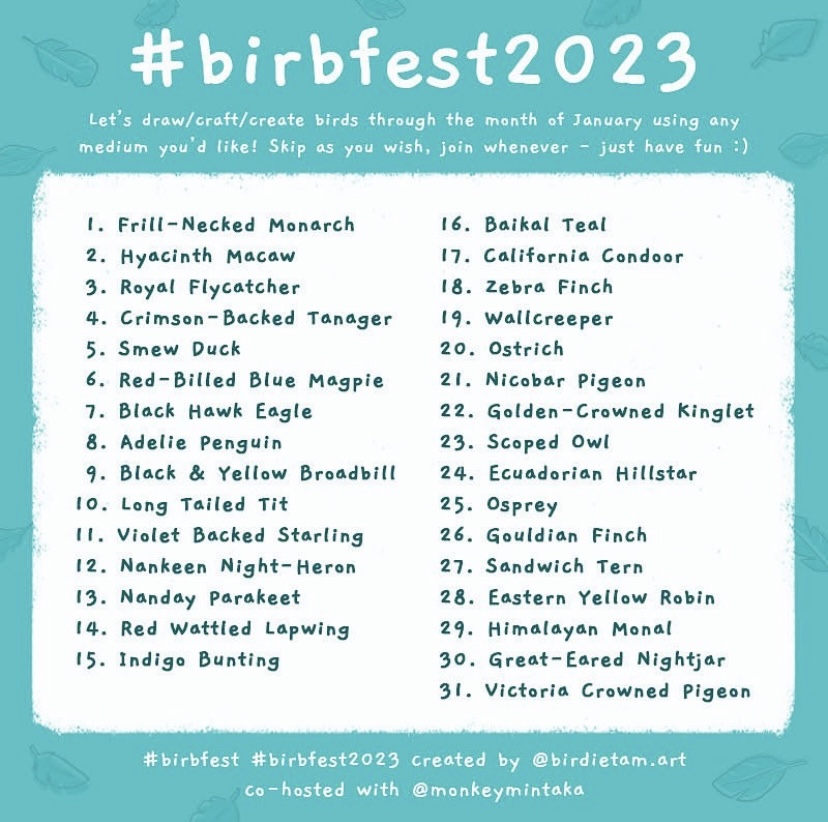The image is an advertisement for BirbFest2023, featuring a bright teal or turquoise background adorned with delicate leaf outlines. At the top, white text prominently displays the event's name, "BirbFest2023," followed by an invitation: "Let's draw, craft, create birds through the month of January using any medium you'd like. Skip as you wish, join whenever, just have fun!" This cheerful message is accentuated with a smiley face. A large white rectangle in the middle contains a handwritten-style font in darker turquoise or black, listing 31 bird species to be illustrated throughout January. These include the Frilled-necked Monarch, Hyacinth Macaw, Royal Flycatcher, Crimson-backed Tanager, Smooth Duck, Red-billed Blue Magpie, Blackhawk Eagle, Adderley Penguin, Ostrich, Scops Owl, and many more. At the bottom, smaller hashtags: #BirbFest and #BirbFest2023, along with credits confirming the event was created by @birdytam.art and co-hosted with @monkeymintaka.